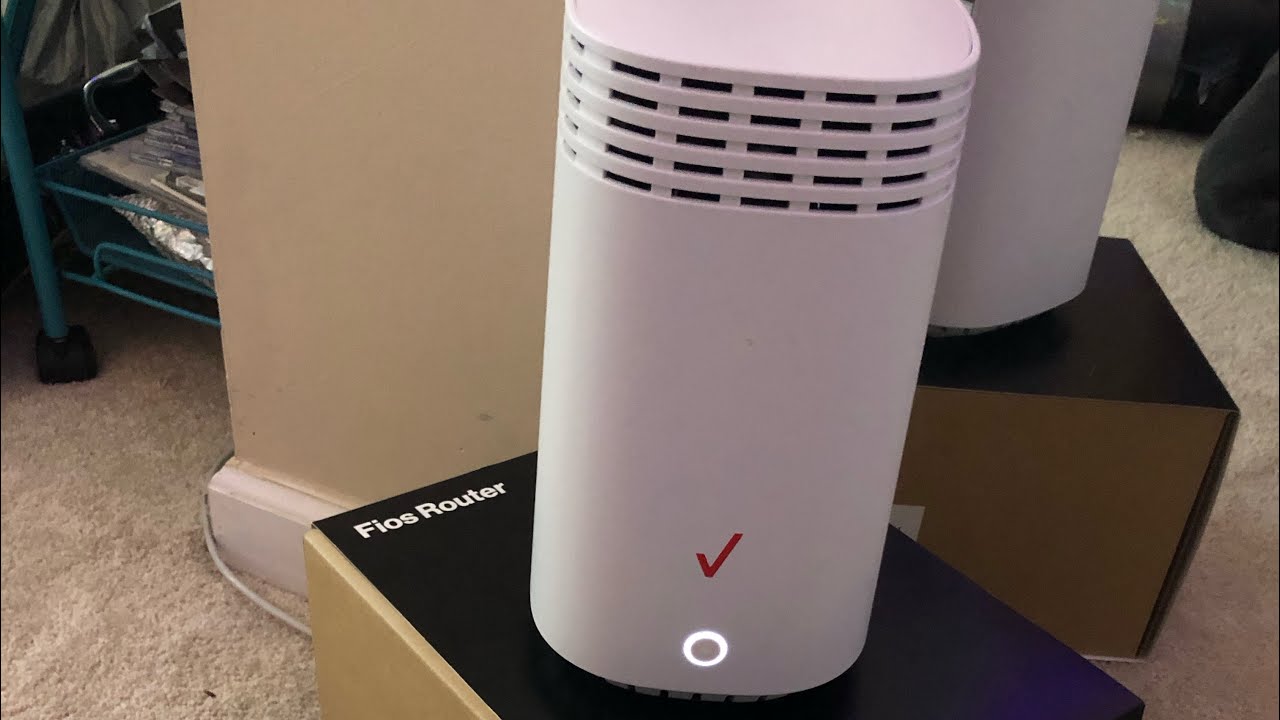The image depicts a large, white cylindrical internet router with vent holes at the top, positioned on a black and tan box labeled "Fios Router." A prominently glowing white button with a red checkmark is visible on the front of the router. The scene appears to be indoors, in a house with tan carpeting, next to a tan wall. To the right, another identical router and box setup is partially visible in what seems to be a reflection in a mirror. There is also a plain box behind which a blue basket containing a piece of white paper is noticeable. Additional details include a glimpse of a bluish bed frame to the left, a black pillow on the right, and a white cord on the floor. The area around the router has a cluttered feel, with various household objects scattered about.